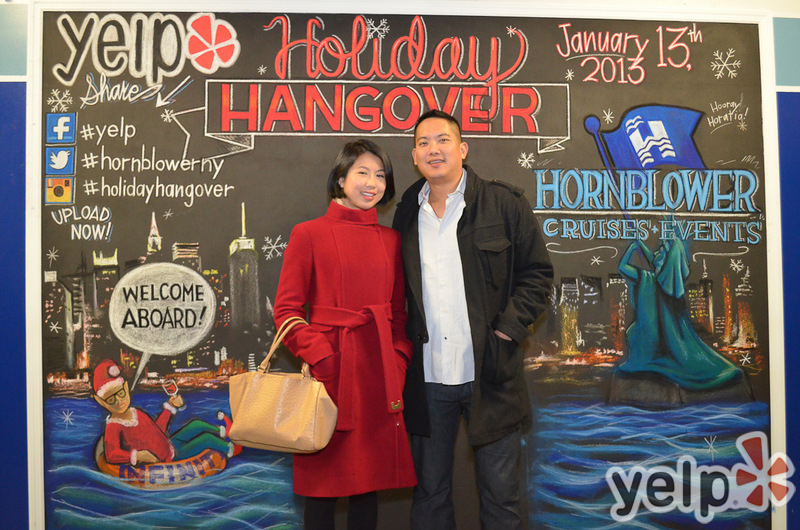This is a color photograph of a young Asian couple posing in front of a large poster. The woman, on the left, is wearing a closed long red coat and holding a brown handbag. She has black hair and is dressed in black pants with her hands in her pockets. To her right stands a man with short black hair, clad in a black jacket over a collared blue shirt and dark pants. Both are smiling. The poster behind them prominently displays "Holiday Hangover" in red text, with event details like "January 13, 2013" and phrases such as "Welcome Aboard" and "Upload Now." The poster is also branded with the Yelp logo and Hornblower Cruise Events logo featuring a blue flag. In the background, the nighttime New York City skyline is visible, along with the Statue of Liberty and a man in a Santa costume floating on a river.